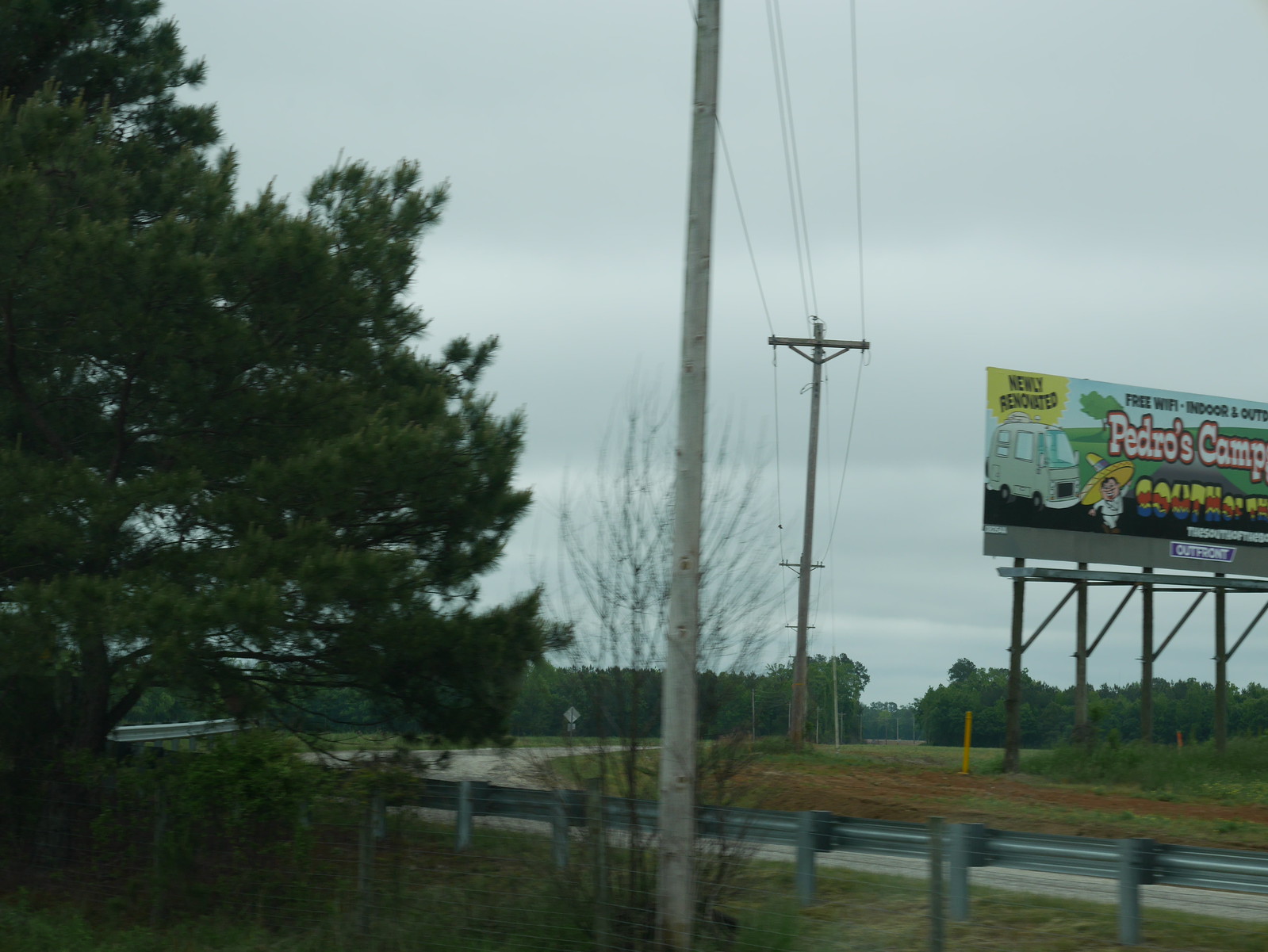A photograph captures a serene outdoor scene from a wooded area adjacent to a small cement road. The image presents the backside of a guardrail, partially shielding a field from the road. In the field, a person stands, giving a sense of scale and human presence against the natural surroundings. The road, narrowly visible beyond the guardrail, is flanked by expanses of grass and dotted with tall trees that stretch towards the back of the frame, creating a lush green backdrop. On the right side of the image, a prominently placed billboard advertises "Pedro's Camp," showcasing an inviting RV and a cheerful man dressed in a white suit and sombrero. The billboard's text, which includes a note about being "newly renovated," suggests it's promoting a rejuvenated campground, hinting at leisure and adventure opportunities.